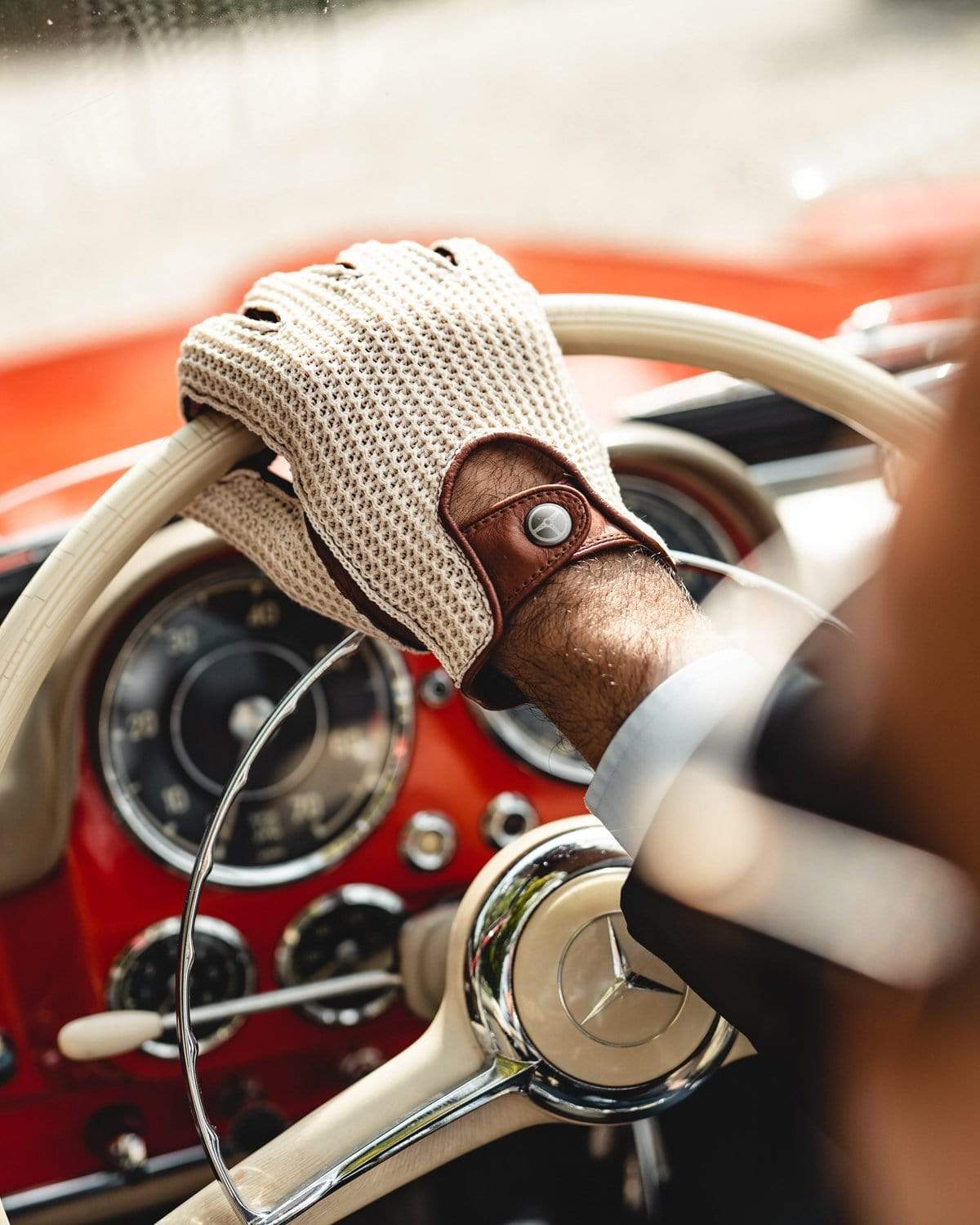This photograph captures a photo-realistic interior of a classic Mitsubishi vehicle, focusing on a close-up of a driver's hand gripping the top of a cream white leather steering wheel adorned with a triangle silver Mitsubishi logo. The driver's hand, covered in a white cloth glove with a leather latch in the center, exudes a vintage elegance, possibly hinting at an advertisement for luxurious driving gloves. In the background, partially blurred, is a vibrant red dashboard with out-of-focus circular gauges and various control buttons. The upper part of the image reveals the red hood of the car and a section of the windshield, further accentuating the classic and stylish ambiance. The slight glimpse of the man's glasses and part of his face adds a subtle yet human touch to the scene.